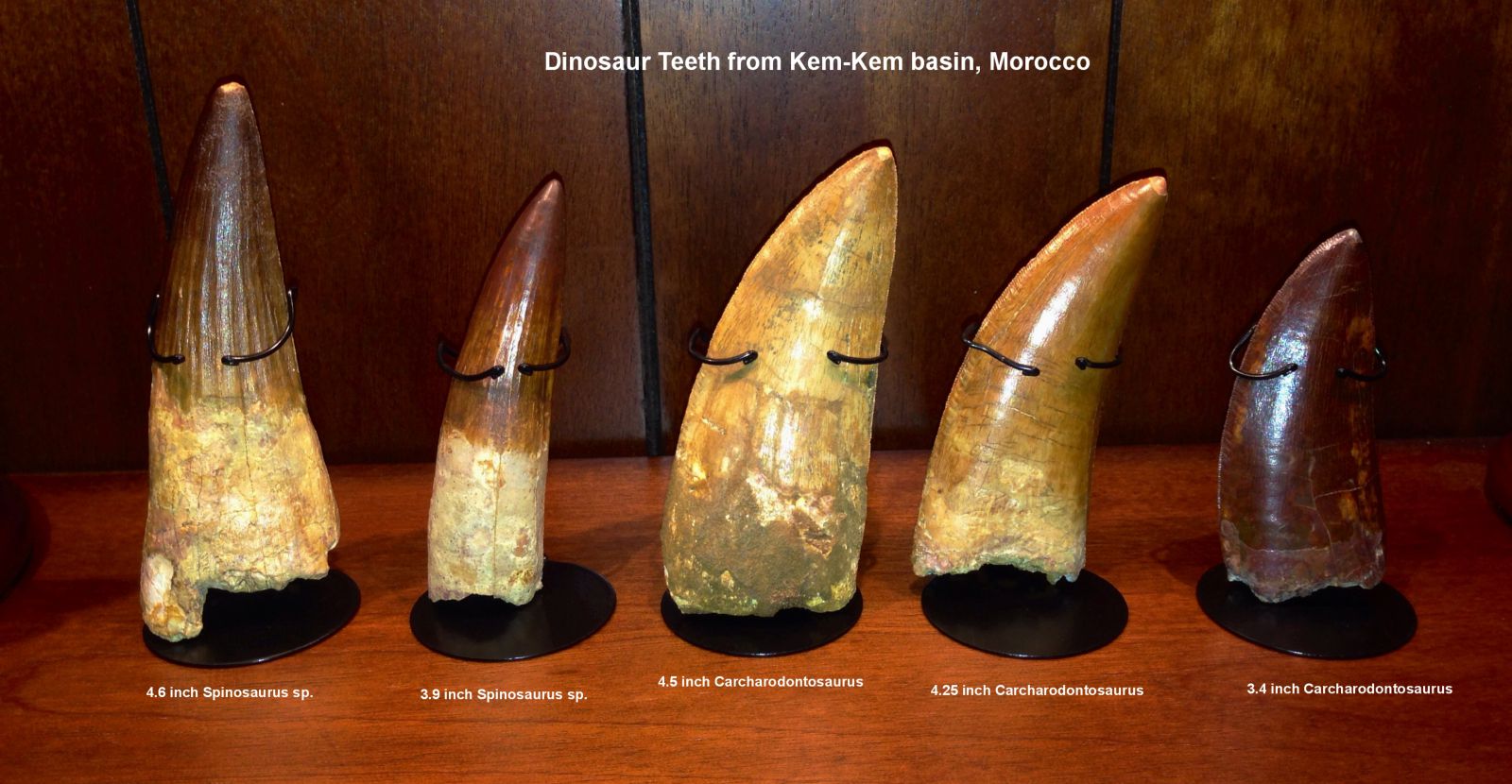This detailed photo showcases an exhibit of dinosaur teeth from the Kem Kem Basin in Morocco, displayed in a dark wooden cabinet with paneling. Positioned beneath a white overlay title that reads "Dinosaur Teeth from Kem Kem Basin, Morocco," the exhibit features five distinct teeth. 

Starting from the left, the first tooth is a 4.6-inch Spinosaurus specimen with a darker brown tip transitioning to a beige base. Next to it, a narrower 3.9-inch Spinosaurus tooth exhibits a shiny brown tip and an ivory bottom. 

The middle tooth belongs to a Carcharodontosaurus, measuring 4.5 inches, and is characterized by a broader, more massive shape with a consistent brownish-beige color. Following this is a 4.25-inch Carcharodontosaurus tooth with a more pronounced angle and a deeper brown hue. 

The final tooth on the right is a shorter, stouter 3.4-inch Carcharodontosaurus, distinguished by its dark brown coloration, almost appearing red, and a shape reminiscent of a shark tooth. Each tooth details its length and dinosaur type in white text at the bottom, enhancing the visual and educational impact of the exhibit.